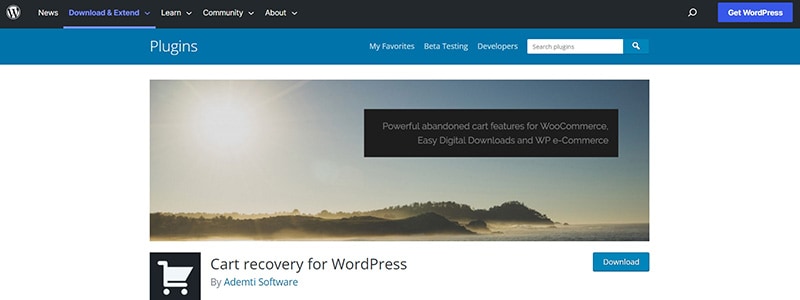The image is a screenshot from a world news webpage. At the very top, there is a black strip featuring a white circle with a black "W" inside it, followed by the word "news" in white. Adjacent to this, there are blue text links that read "Download" and "Extend," separated by a blue line. The white text links "Learn," "Community," and "About" are found next. On the far right, there is a white magnifying glass icon and a smaller blue text box saying "Get WordPress" in white.

Beneath the black strip, a larger blue text box with the word "Plugins" in white letters is visible. This is followed by white text links that say "My Favorites," "Beta Testing," and "Developers," alongside a white search bar marked "Search plugins," with an accompanying white magnifying glass icon.

The main background below is white, featuring a prominent beach scene. Overlaid in the upper right-hand corner of this scene is a black text box stating, "Powerful abandoned cart features for WooCommerce," followed by "Easy Digital Downloads" and "WP eCommerce" in white letters. Below this, there is a black square containing a white shopping cart icon, adjacent to the black text, "Cart recovery for WordPress." The word "Buy" appears in black next to the software name "Dematy Software" in blue. On the right-hand side, a small blue box with "Download" in white lettering is present.